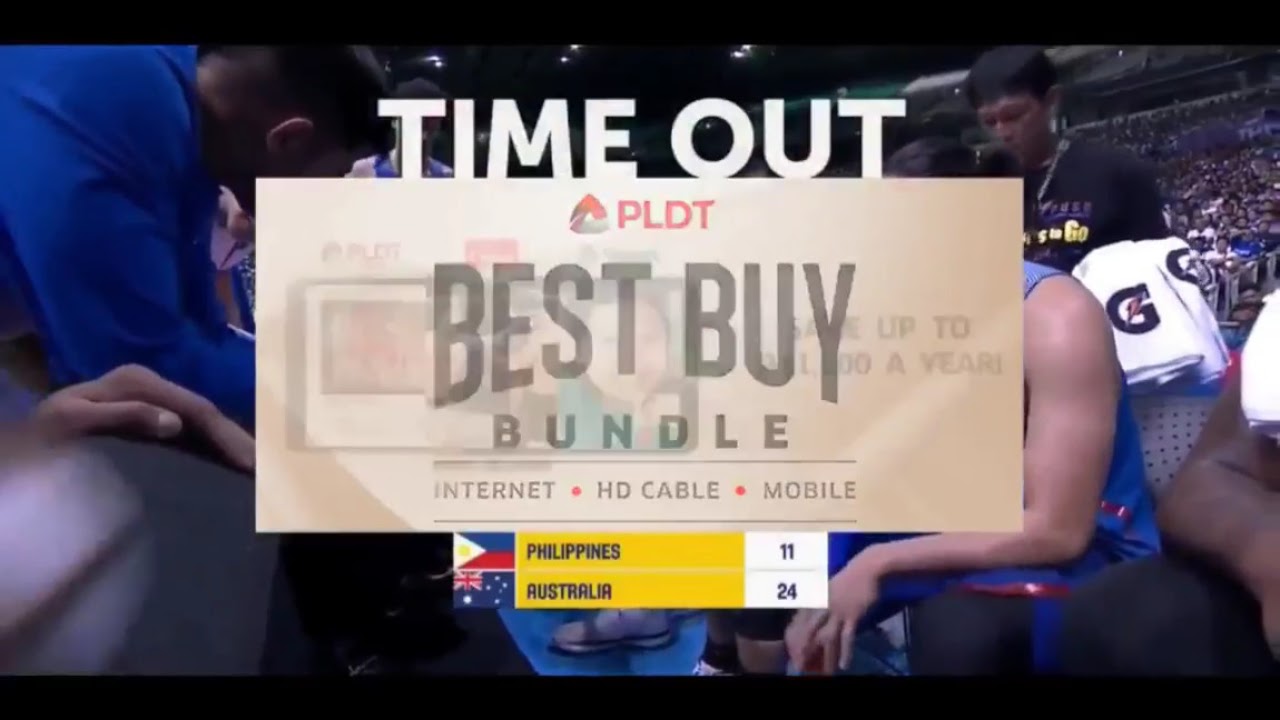The image is a detailed screenshot of a commercial overlaid on a sports event photograph. The background shows players in a stadium, likely from a basketball game, surrounded by a large crowd seated in a raised stairway area. The overlay consists of multiple elements: at the top, the capitalized text "Time Out" is prominently displayed in off-white. Beneath this, there is a tan rectangle with faded black edges, containing the text "Best Buy Bundle" followed by the words "Internet," "HD Cable," and "Mobile" listed underneath. Below this rectangle, another thinner horizontal section presents the flags and scores of two teams: the Philippines with a score of 11, and Australia with a score of 24. The image is horizontal and framed by thin black stripes at the top and bottom.